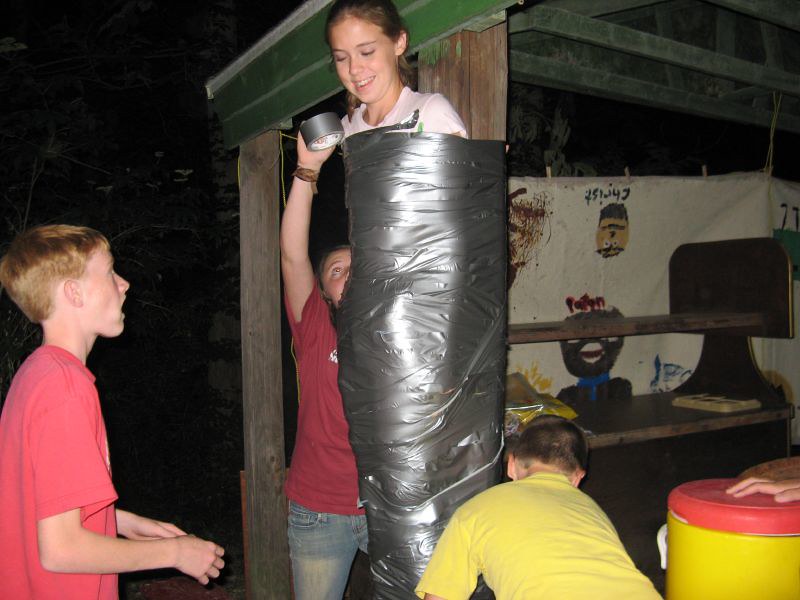This nighttime outdoor photograph captures a humorous scene involving several children and a playful use of duct tape. In the center, there is a smiling young girl with brown hair, wearing a white t-shirt, who is completely wrapped in duct tape from her collarbone down to a brown pole. Positioned behind her is another child, potentially a girl, wearing a red shirt and blue jeans, holding a roll of duct tape up to the taped girl's shoulder. To the left, a boy with short blonde hair is also wearing a red shirt, looking attentively at the girl who is duct-taped. Towards the bottom center, another child in a short-sleeved yellow shirt is bending over, seemingly taping the girl’s feet. The backdrop on the right features a white tapestry decorated with faces and flanked by two vertical wooden boards, resembling a carnival game setup. The image suggests a spontaneous and lighthearted moment, with the taped girl’s broad smile indicating that she is enjoying the playful situation.